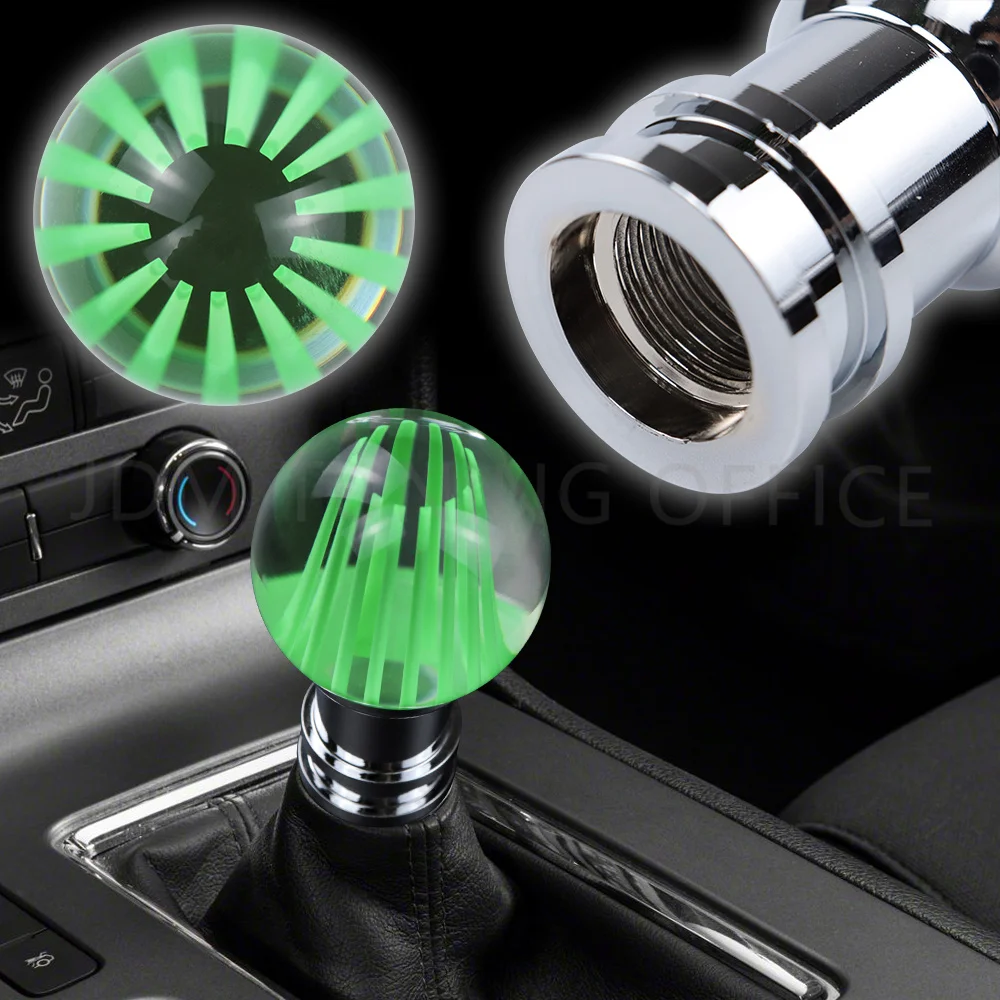The image captures the detailed interior of a car with a prominent gearshift being the focal point. The gearshift is unique, featuring a translucent green ball with green lines inside and a black center, and is silver around the shifting mechanism. This gearshift is highlighted by a separate, close-up view in the upper left corner, showcasing its detailed design and resemblance to an eye, with the added feature that looks like it could be screwed on. The background of the car interior is predominantly black, with silver accents around various controls. On the left of the gearshift, an air-cooling button with right-facing arrows is situated above a temperature control knob marked with blue (cold) on the left and red (hot) on the right, which also includes some black buttons nearby. The right side of the image is mostly blacked out, showing a black seat. Also mentioned is a possible cigarette lighter hole, indicating further typical car interior elements. The upper right portion of the image shows details resembling the gearshift's socket, with semi-transparent text reading something with "office" in the middle.